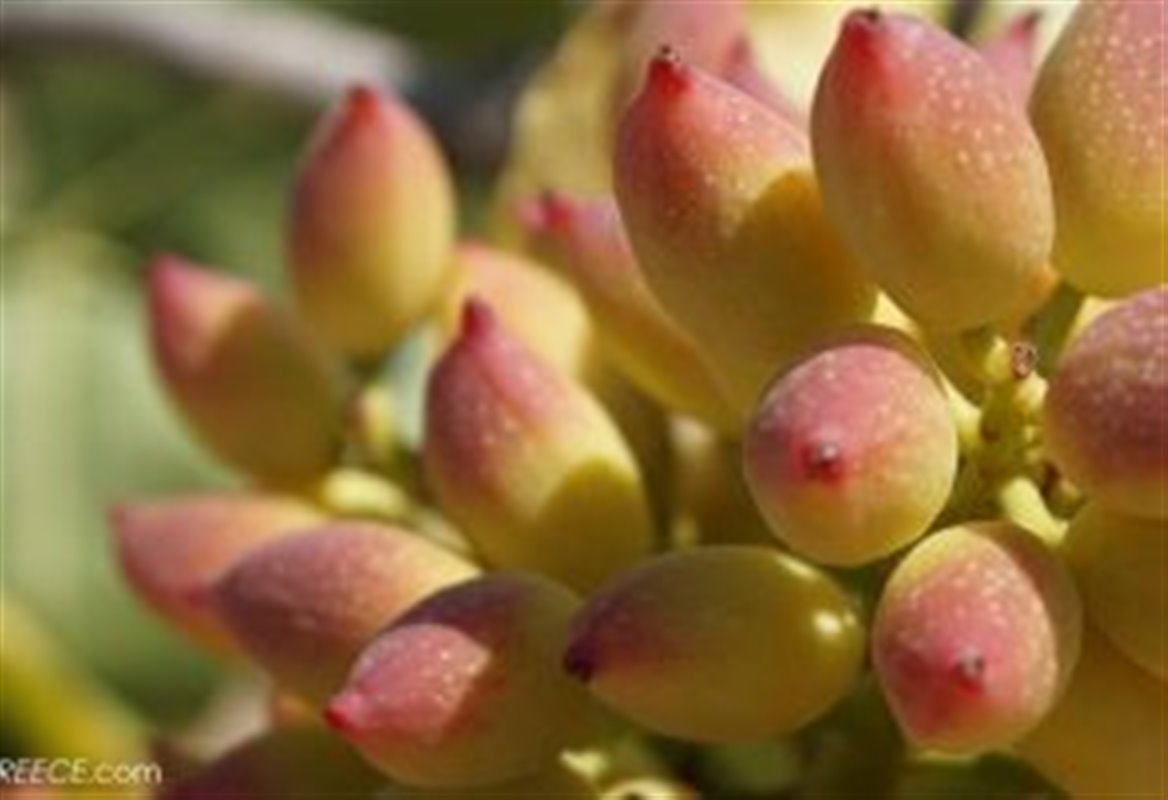This up-close photograph captures a tight bunch of elongated pods resembling grapes, growing from stems matching their green hue. Each pod is green, gradually dusted with a rosy pink hue towards the tips, giving them a striking appearance. The photograph is sharply focused on the pods, blurring out the background into a palette of medium greens, suggestive of surrounding foliage. In the lower left-hand corner of the image, the text reads "reese.com." The image highlights the textures and colors of the pods, from the green base to the pink-tinted tips, making it visually rich. Despite the slight blur and overall poor quality mentioned, the photograph prominently showcases the distinctive, pointy-ended pods against their leafy backdrop.